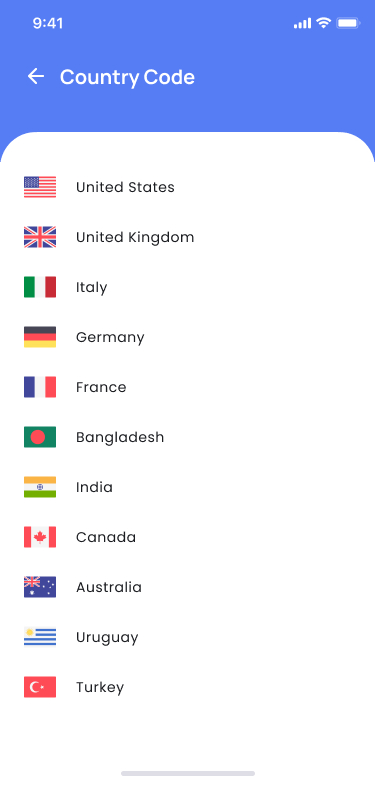This is a detailed caption for the provided description:

---

A mobile phone screenshot captured at 9:41 AM, displaying a strong signal, strong WiFi connection, and a fully charged battery. At the top left, an arrow pointing to the left is labeled "Country Code" in white text on a blue background. Below this, a list of countries is displayed, each with its respective flag and name. The countries and their flags are as follows: 

- United States 🇺🇸
- United Kingdom 🇬🇧
- Italy 🇮🇹
- Germany 🇩🇪
- France 🇫🇷
- Bangladesh 🇧🇩
- India 🇮🇳
- Canada 🇨🇦
- Australia 🇦🇺 
- Uruguay 🇺🇾
- Turkey 🇹🇷

A grey line divides the screen horizontally, all set against a white background. The country names are in black text, and the flags are presented in their respective native colors.